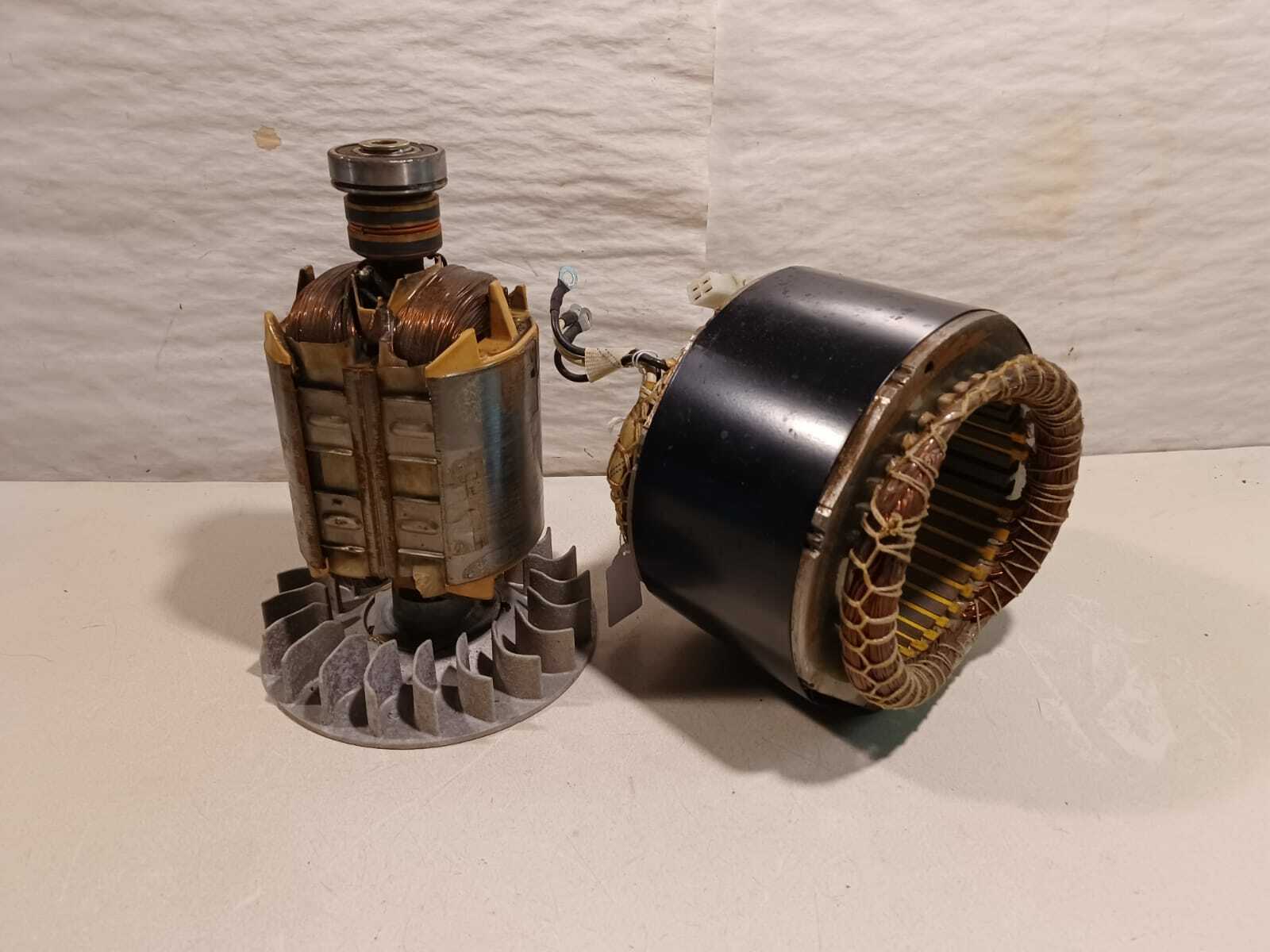The photograph showcases two vintage devices placed against a rough, light gray background with a crinkle-paper texture. The device on the left, which appears to be an upright cylindrical apparatus, is constructed from bronze and gray metal, featuring a base with small, curved structures. At its top, the device transitions into a darker metal capped area, enclosing coiled copper wire. The device on the right is a round, black-and-silver metallic object, outlined by a ring of copper wire. It has a white paper tag attached to it and two black cords extending from its back. The layout suggests the possibility that the device on the right may connect to the one on the left. A subtle brown stain on the left and a streak on the right edge of the background add to the aged appearance of the scene.